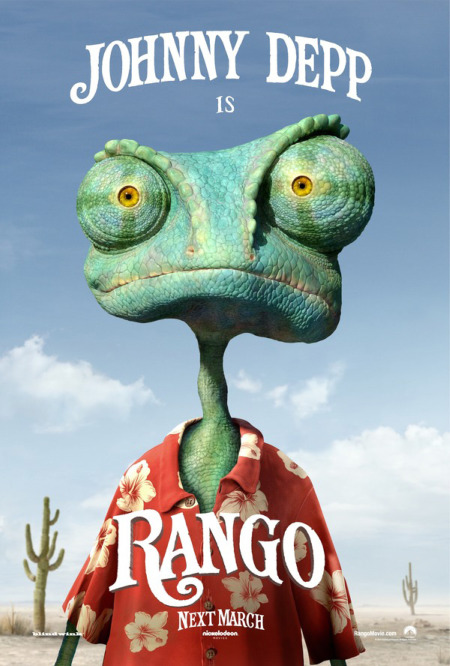The promotional poster for the animated film "Rango" showcases the titular character, Rango, voiced by Johnny Depp. The caption prominently states "Johnny Depp is Rango" with the title "Rango" and the phrase "Next March" indicating the film's release. Paramount and Nickelodeon are credited as the production companies behind the film. The image features Rango, a chameleon, wearing a vivid red Hawaiian shirt adorned with white flowers. He stands in a desert setting characterized by muted blue skies with white puffy clouds, and two cacti—one closer and one farther in the distance—frame the background. Rango is depicted with large, expressive yellow eyes, a long neck, and a distinctly human-like posture, standing on his hind legs. Despite the comedic and slightly perplexed expression on his face, the poster effectively conveys the film's slightly comedic animated take on Western tropes.